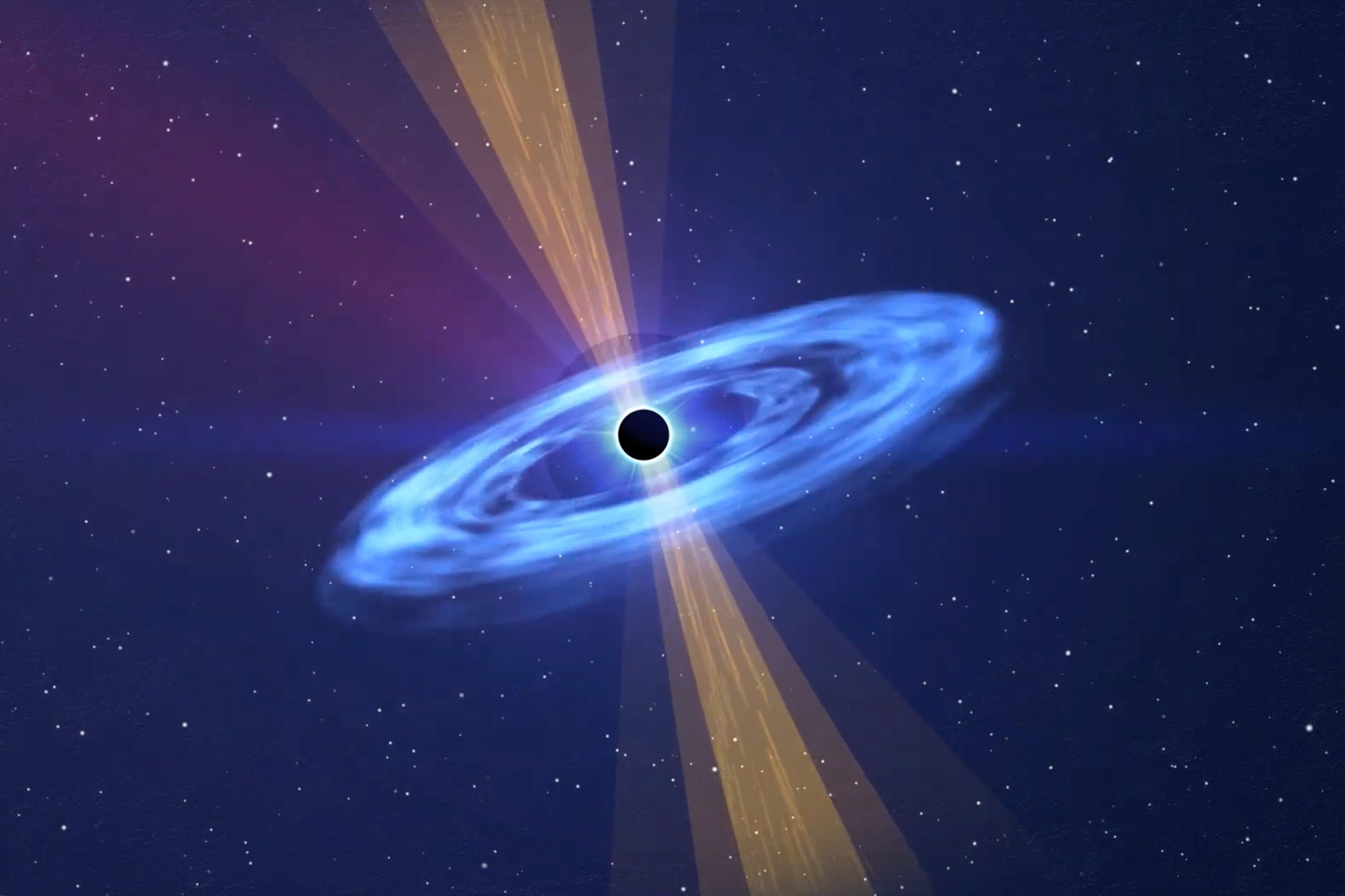This highly detailed illustration, resembling a computerized render, captures a mesmerizing outer space scene. Set against a backdrop that transitions from a deep blue to black on the edges, the sky is sprinkled with countless white specks, resembling a starry night. In the center of the image, a small, pitch-black circle, possibly representing a black hole, emanates a sense of cosmic mystery. Encircling the black hole is a bright, glowing ring, giving it an appearance similar to a solar eclipse.

Radiating from the black circle, a flat, light blue wave of light expands diagonally, reminiscent of Saturn’s rings, extending halfway across the image. Accentuating the dramatic impact of the central black hole, yellow rays of light shoot out from the top and bottom, angling slightly to the left, creating a dynamic sense of movement. The entire composition is illuminated by vivid colors, with a subtle but noticeable purple glow enhancing the otherworldly atmosphere. The illustration vividly captures the awe-inspiring beauty and complexity of the cosmos.